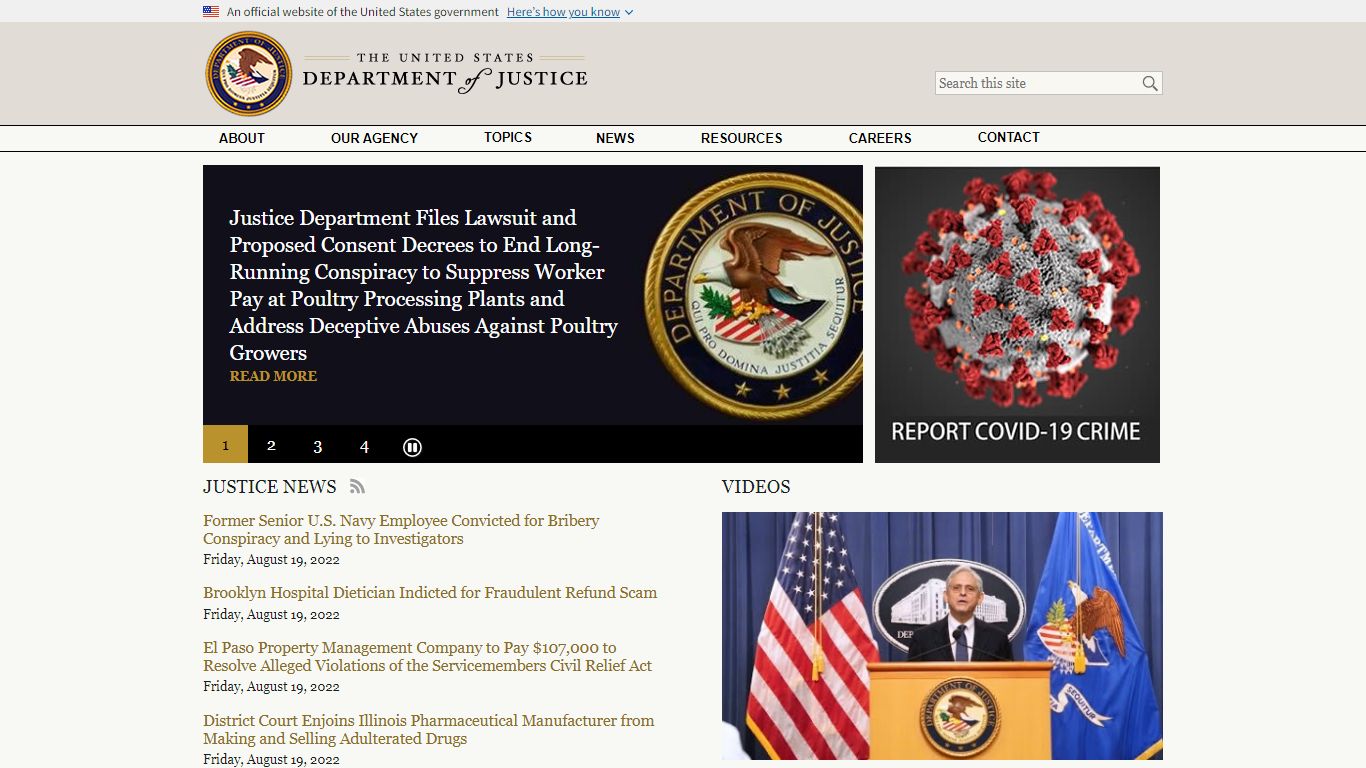The image features a webpage from the United States Department of Justice's official website. At the very top of the page, a blue underlined text states, "An official website of the United States government. Here's how you know," accompanied by a pull-down menu.

Prominently displayed in black text on a gray background to the left is the title, "United States Department of Justice," next to the department's seal. To the right, there is a search bar with a magnifying glass icon for site searches.

Below the header, a navigation band includes tabs labeled: "About Our Agency," "Topics," "News," "Resources," "Careers," and "Contact." Underneath this band, there is a section on the left side with a black background and white font, featuring the Department of Justice emblem, which includes the motto "Quid Pro Quo Domina, Justia Secura" encircling an eagle.

The main headline reads, "Justice Department files lawsuit and proposed consent decrees to end long-running conspiracy to suppress worker pay at poultry processing plant and address deceptive abuses against poultry growers." A "Read more" link is highlighted in an orangey-yellow color. 

At the bottom of the section, pagination icons numbered 1 to 4, with the first number highlighted in gold, and a circular pause button with two vertical lines, are visible. Below them, a section titled "Justice News" is indicated, followed by introductory text regarding a former senior U.S. Navy official.